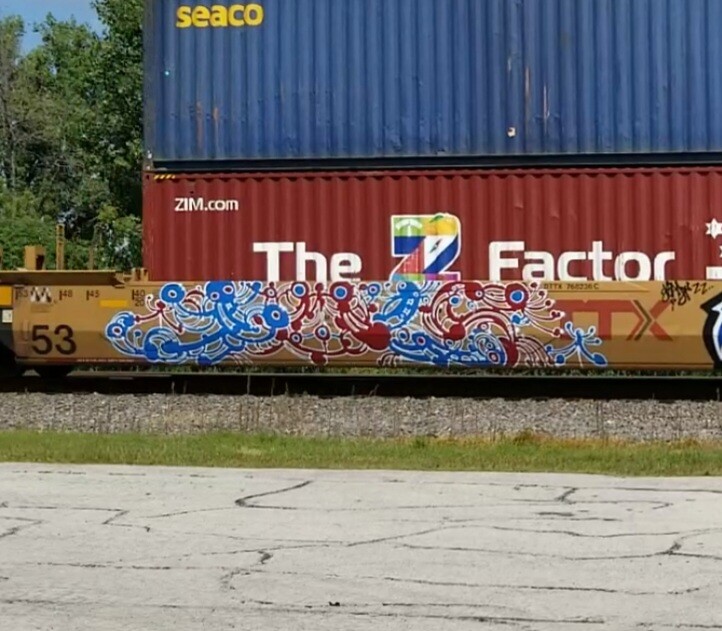This photograph captures a straight-on eye-level view of a weathered rail car chassis, which bears two large, stacked steel shipping containers. The bottom container is red and adorned with abstract blue and red graffiti, featuring swirls, dots, and eye motifs. It prominently displays the text "the Z factor" in white, with a multi-colored, stylized 'Z', and the URL "Zim.com" in the upper left corner. The top container is blue, marked with the word "Seaco" in yellow text in its upper left corner. The rail car itself is framed by a road at the bottom of the image, marked with streaks of tar from previous patch jobs, and a strip of slightly dry grass. In the distant top left of the photo, several trees can be seen.